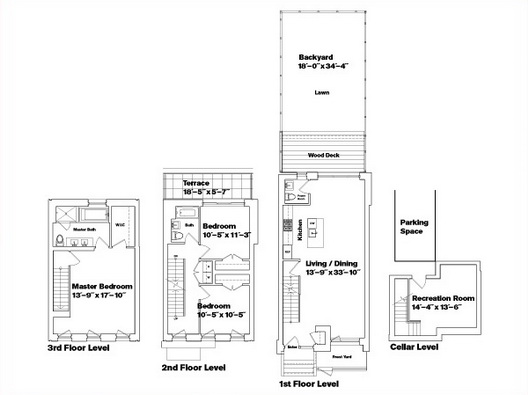This floor plan consists of a four-level home, with each level meticulously laid out side by side from left to right. The levels are labeled as follows: cellar level, first floor level, second floor level, and third floor level.

Starting with the **cellar level**, we find a recreation room accompanied by stairs that descend into this space. Additionally, a dedicated parking area is drawn in, illustrating its convenience and accessibility.

Moving to the **first floor level**, which is significantly more elongated vertically, we observe a backyard area and a wood deck. Within the indoor space, there is a kitchen, a combined living and dining room, and a modest bathroom equipped with a toilet and a sink. The front of this floor features an exterior staircase leading to what appears to be a balcony, enhancing the entrance's aesthetic appeal.

Adjacent to this is the **second floor level**, which accommodates two bedrooms and a bathroom. The bathroom is furnished with a toilet, sink, and bathtub. The dimensions of the bedrooms are precisely 10 feet 5 inches by 11 feet 3 inches, and 10 feet 5 inches by 10 feet 5 inches, respectively. The space also includes closets nestled between the two bedrooms and a staircase connecting to the lower level.

Lastly, the **third floor level** is dedicated to the master suite. The master bedroom itself is impressively spacious, measuring 13 feet 9 inches by 17 feet 10 inches. The layout includes an ensuite bathroom featuring a tub and shower, a toilet, and dual sinks. Additionally, a walk-in closet provides ample storage. The stairs from the lower floor seamlessly connect to this luxurious and private retreat.

This detailed and thoughtfully designed floor plan illustrates a harmonious blend of functional and aesthetic elements across all four levels of the home.